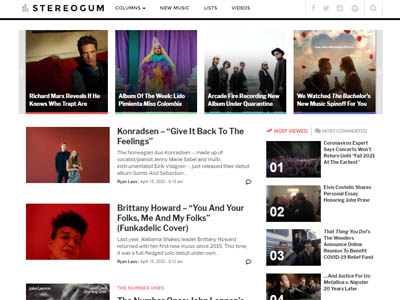The image appears to be a screenshot of a computer displaying the Stereo Gum website. At the very top, the website's name "Stereo Gum" is prominently displayed in black. To the right of the title, there are four navigational options: "Columns," "New Music," "Lists," and "Videos."

Below the navigation bar, there are four square thumbnails arranged horizontally. The first thumbnail features a man sitting in a dimly lit room on a red sofa. The second thumbnail displays a woman with long blonde hair and is labeled "Albums of the Week." The third thumbnail portrays a musical group standing on a beach. The fourth and final thumbnail shows a man and a woman with a sky backdrop, where the clouds are artistically shaped into a heart.

Further down the page, there are two headlines in the central part of the screen. The first headline reads "Conradson, Give It Back to the Feelings," accompanied by a picture on the left featuring a red background with a man and a woman. The second headline is titled "Brittany Howard: You and Your Folks, Me and My Folks (Funkadelic Cover)," with an image that shows a person with black hair and glasses set against a predominantly red background. The text of another headline is partially visible at the bottom of the screen but is cut off.

This detailed description provides a comprehensive overview of the key visual elements present in the screenshot of the Stereo Gum website.